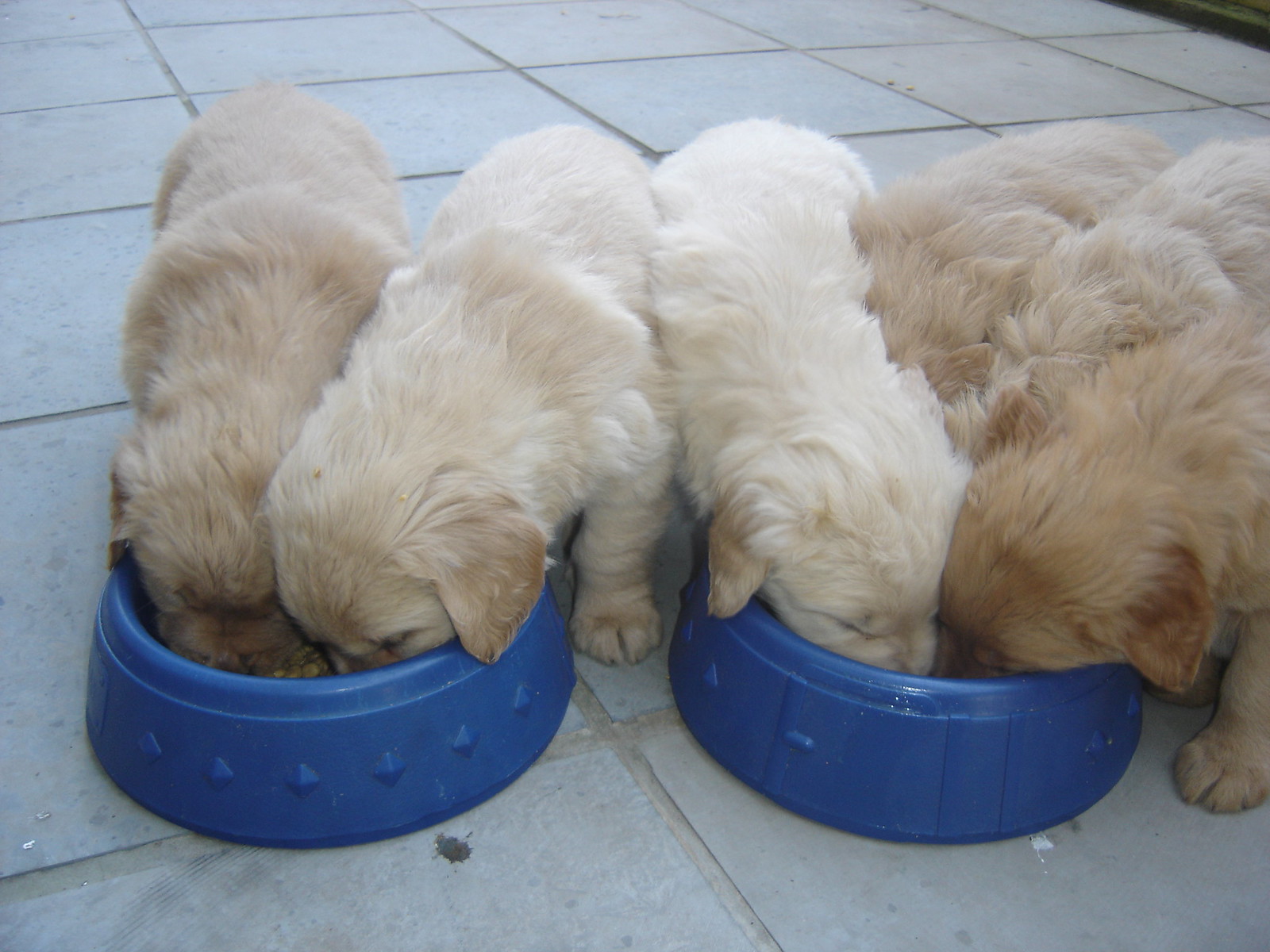The image showcases six energetic golden retriever puppies, all approximately eight to ten weeks old, eagerly eating from two bright blue dog bowls placed on a white tile floor, presumably in a kitchen. The bowl on the left side of the image is accompanied by two light-colored puppies with almost white fur. On the right side, four puppies with varying shades of golden fur, from lighter to darker browns, crowd together, their heads buried in the bowl as they eagerly consume their food. All puppies are standing on their four tiny paws, creating an adorable, chaotic scene of mealtime urgency. A small detail includes a dead bug, possibly a beetle, lying on the floor, adding a touch of realism to this charming, candid moment.